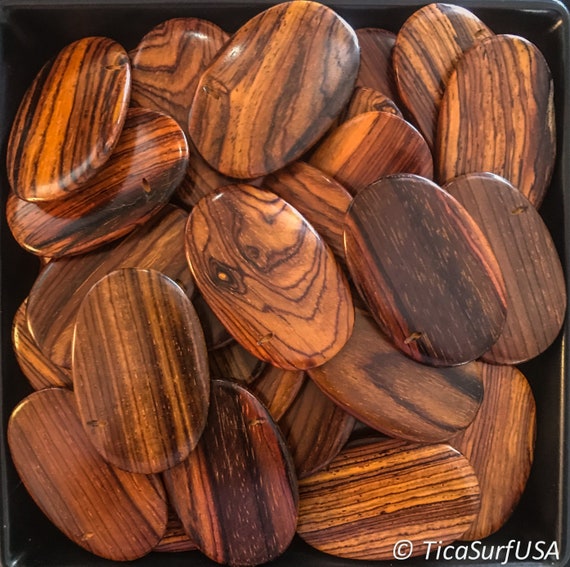This photograph features a collection of polished, oval-shaped wooden pieces, neatly piled together inside a square, black plastic bucket. The wooden ovals exhibit various natural grains and colors, enhancing their aesthetic appeal. One notable piece in the foreground is mainly tan with a distinctive black line resembling the head of a cat. Another piece stands out with its lighter brown edges and a dark, almost black center. In the bottom right corner of the image, the text “TICA Surf USA” is visible, along with a copyright symbol, suggesting a possible connection to a surf shop or surf-related products. The overall scene presents approximately twenty such wooden pieces, each carefully crafted and visually pleasing, though their precise purpose remains unclear.